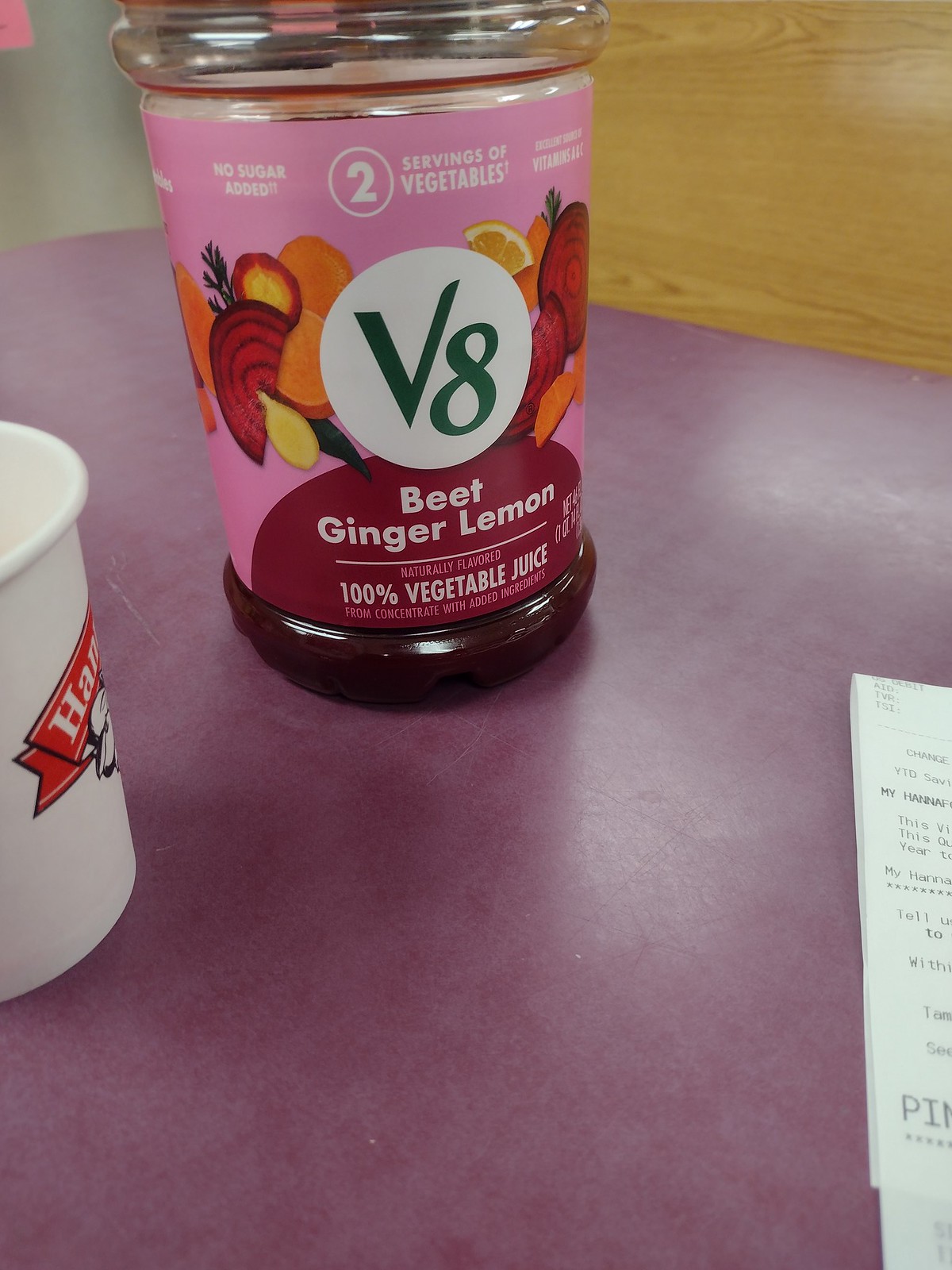In the image, there is a photograph of a table whose location is ambiguous—it could be in a kitchen or perhaps in a restaurant. The table has a smooth, purple tabletop. Behind the table, there is a booth-style seat with a long wooden backrest. On the table, prominently placed in the center, is a bottle of juice. The bottle is clear and purple, labeled "V8 Beet Ginger Lemon 100% Vegetable Juice." To the left of the bottle, there is a small paper cup bearing an indiscernible logo. On the right side of the table, partially visible, is what appears to be half of a receipt, suggesting that this setting might be within a restaurant or store.